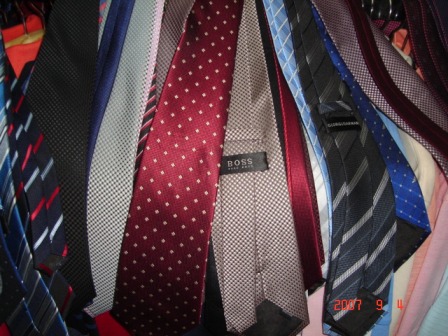The image showcases a large, slightly disorganized stack of around 30 men's ties, held together from the top and cascading down, appearing bunched and mixed. Among the ties, which vary in colors, patterns, and widths, several distinctive ones stand out. In the center, there is a striking maroon tie with white polka dots, and next to it, another eye-catching piece featuring a beige fabric with a black crisscross pattern and the Hugo Boss logo. The ties encompass a diverse palette, including dark red, dark blue, black with silver stripes, light cream with gold and silver polka dots, and even a solid royal blue polka-dotted tie. Notably, there is a mix of patterns, including stripes and digital-style designs in colors like blue, red, gray, and black and white. At the bottom right of the image, the text "2007   9  4" is visible in red letters. Overall, the collection appears vibrant and varied, primarily consisting of Hugo Boss branded ties suitable for suits.